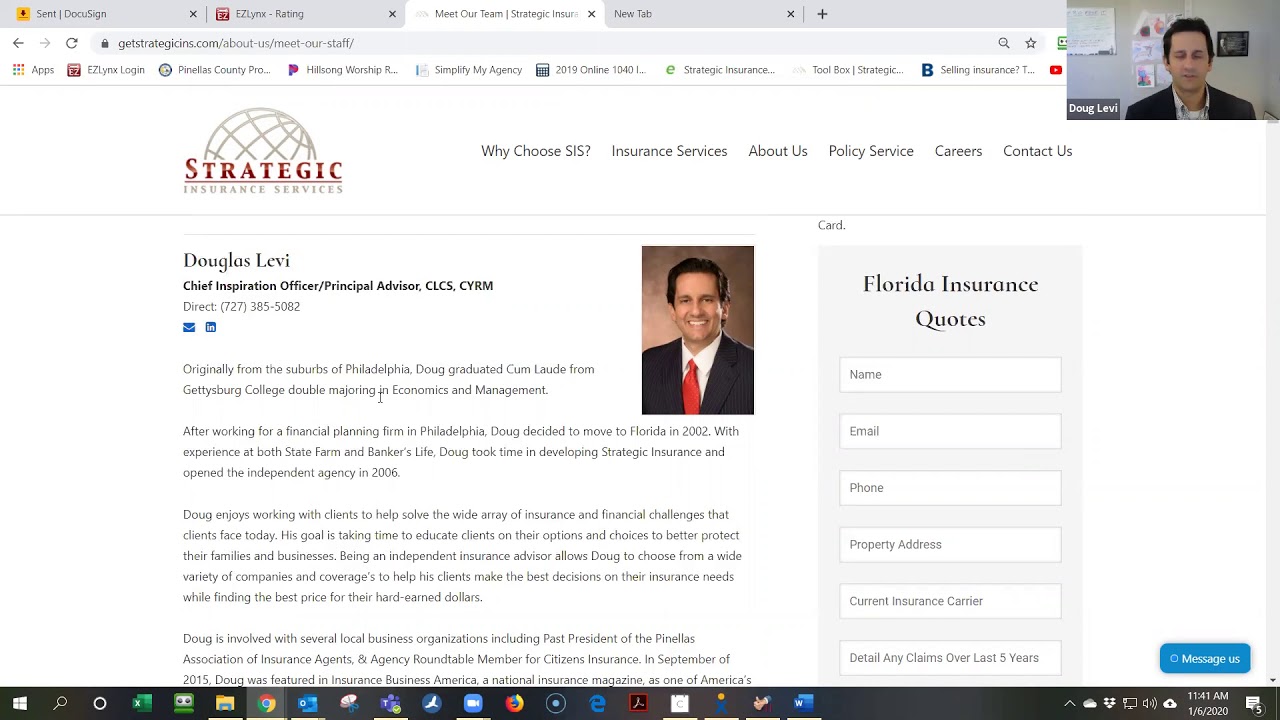The screenshot captures several open browser tabs at the top, including one for DocuSign, Easy Links, and others. The currently visible tab is titled "Meet Our Team" from Strategic Insurance Services. In the upper right corner of the webpage, there's a professional portrait of Doug Levy, a Caucasian man with black hair, dressed in a suit. Below this image, the logo for Strategic Insurance Services is displayed.

The webpage features several navigation links, including "Why Choose SIS?", "Insurance Services," "About Us," "Policy Service," "Careers," and "Contact Us" on the left side. prominently displayed, Douglas Levy is identified as the Chief Inspiration Officer & Principal Advisor with credentials CL CS CY RM. His direct phone number is 727-385-5082.

The description highlights his background, noting he hails originally from the suburbs of Philadelphia. Doug Levy graduated cum laude from Gettysburg College with a double major in Economics and Management. After gaining experience at a financial planning firm in Philadelphia, Doug relocated to Florida in 2002 to further his career.